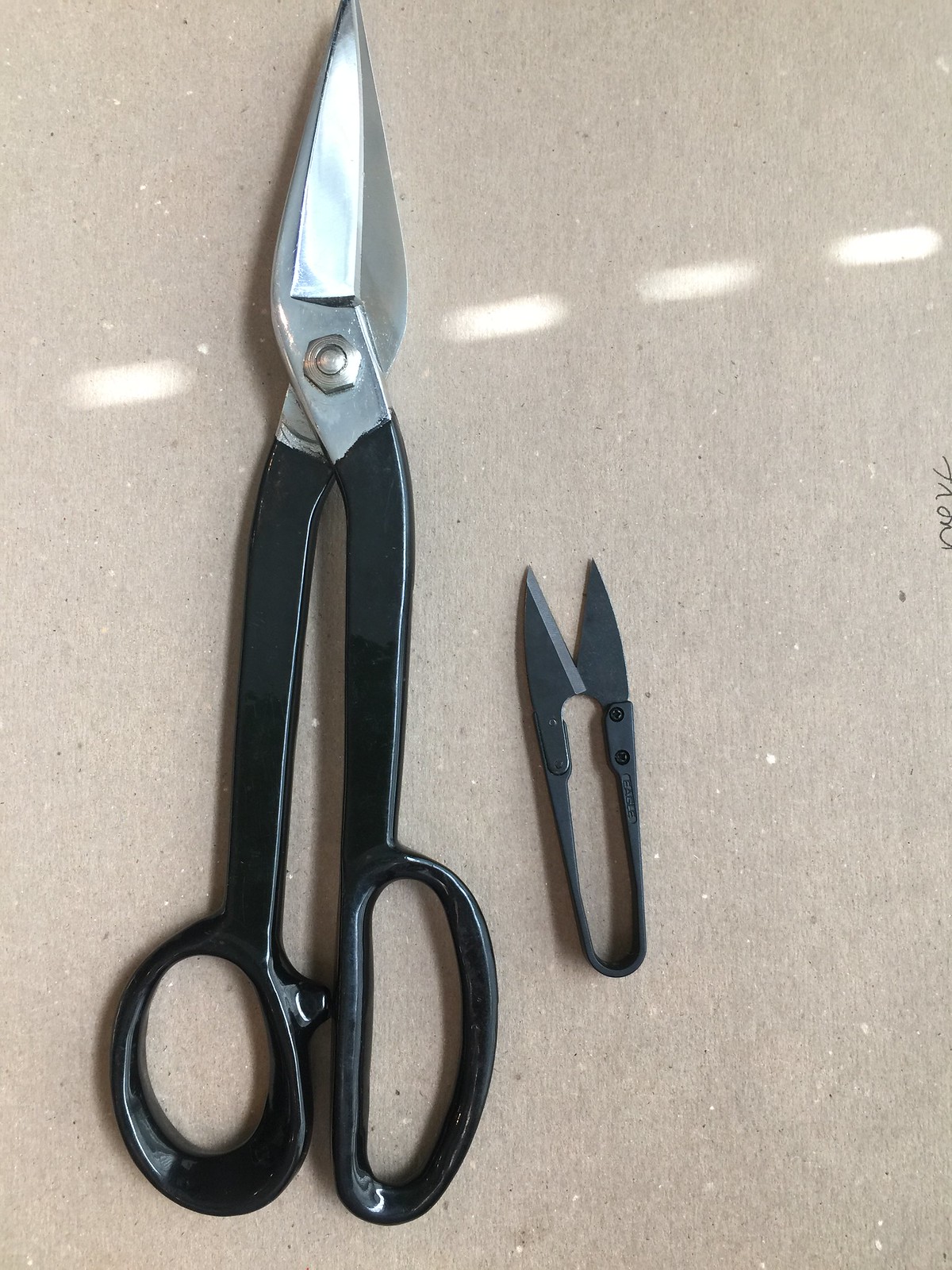This detailed close-up photograph captures two distinct cutting tools displayed on a tan, marble-like countertop. The tool on the left is a pair of long-handled pattern scissors, characterized by their black handles and silver blades. These scissors feature an oval-shaped finger hole with a guard to separate it from the other handle, making it suitable for precisely cutting through fabric patterns. The silver rivet in the middle holds the two parts together, and the black arms extend about an inch and a half into the metal shears.

To the right of the scissors is a smaller U-shaped pair of snips, or nippers, which also have black handles. These snips are designed for precision work, like cutting threads or thin materials, and have two small, sharp blades at the top that curve slightly. The bottom of these snips is rounded, fitting comfortably between the thumb and index finger for easy use.

Both tools are positioned with the handles at the bottom of the image and the cutting parts pointing upwards. Notably, there is some black writing in the right-hand corner of the countertop, which appears to be initials or a small inscription reading "N-E-V-L." The background tan color complements the sophisticated design of these well-crafted tools.